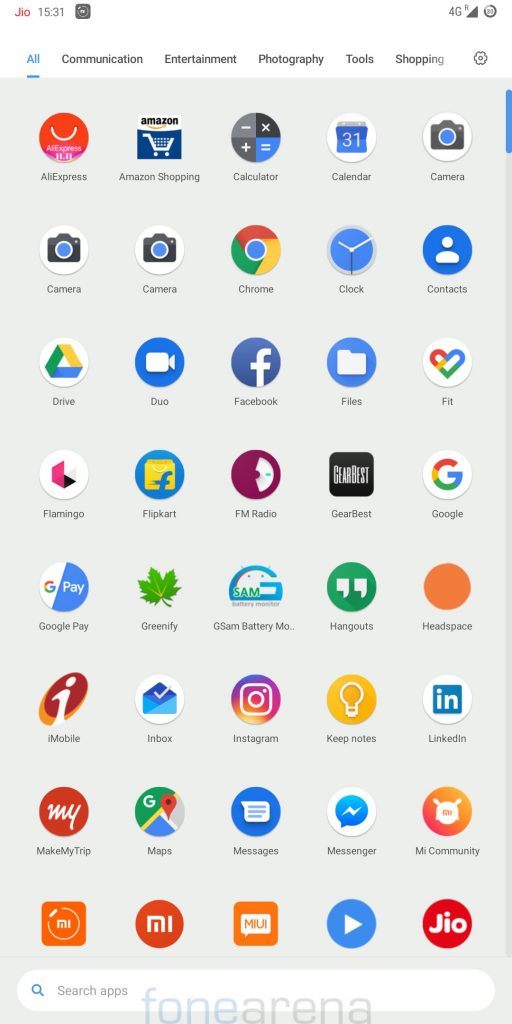This vertical image appears to be a screenshot taken from a smart device, showing a detailed view of its app drawer. The background of the image includes a white glow from the computer screen, making the text and icons more prominent. 

At the top, the status bar displays:
- The "JIO" network in red.
- The time in military format, "1531," in gray.
- Various icons including a 4G triangle indicating the signal strength and a small circular icon.

Below the status bar, the app drawer is categorized with various options, with "All" highlighted in blue and underlined. The other selectable categories are listed in black: "Communication," "Entertainment," "Photography," "Tools," "Shopping," and a "Settings" icon.

The background shifts to a medium gray color, accompanied by a blue scroll bar on the right side, indicating a scrollable list of apps. Each app is represented by a circular icon followed by its respective name underneath.

The visible apps in the screenshot include:
- AliExpress 
- Amazon Shopping
- Calculator
- Calendar
- Camera (repeats thrice)
- Chrome
- Clock
- Contacts
- Drive
- Duo
- Facebook
- Files
- Fit

The next line of visible apps showcases:
- Flamingo
- Flip Art
- Flip Radio
- Gearbest
- Google

Following this, the apps listed are:
- Google Play
- Greenify
- GCM Battery (with truncated text represented by "dot, dot, dot")
- Hangouts
- Headspace

Continuing further, more apps include:
- Mobile
- Inbox
- Instagram
- Keep Notes
- LinkedIn

Additional apps shown are:
- Make My Trip
- Maps
- Messages
- Messenger
- My Community

Further down, the visibility cuts off making only app icons without their names discernable.

At the very bottom, there is a search bar labeled "Search Apps" and a mention of "Phone Arena," possibly indicating a specific section or feature of the app drawer interface.

This meticulous screenshot captures the organized layout and extensive list of apps available on the user's device.